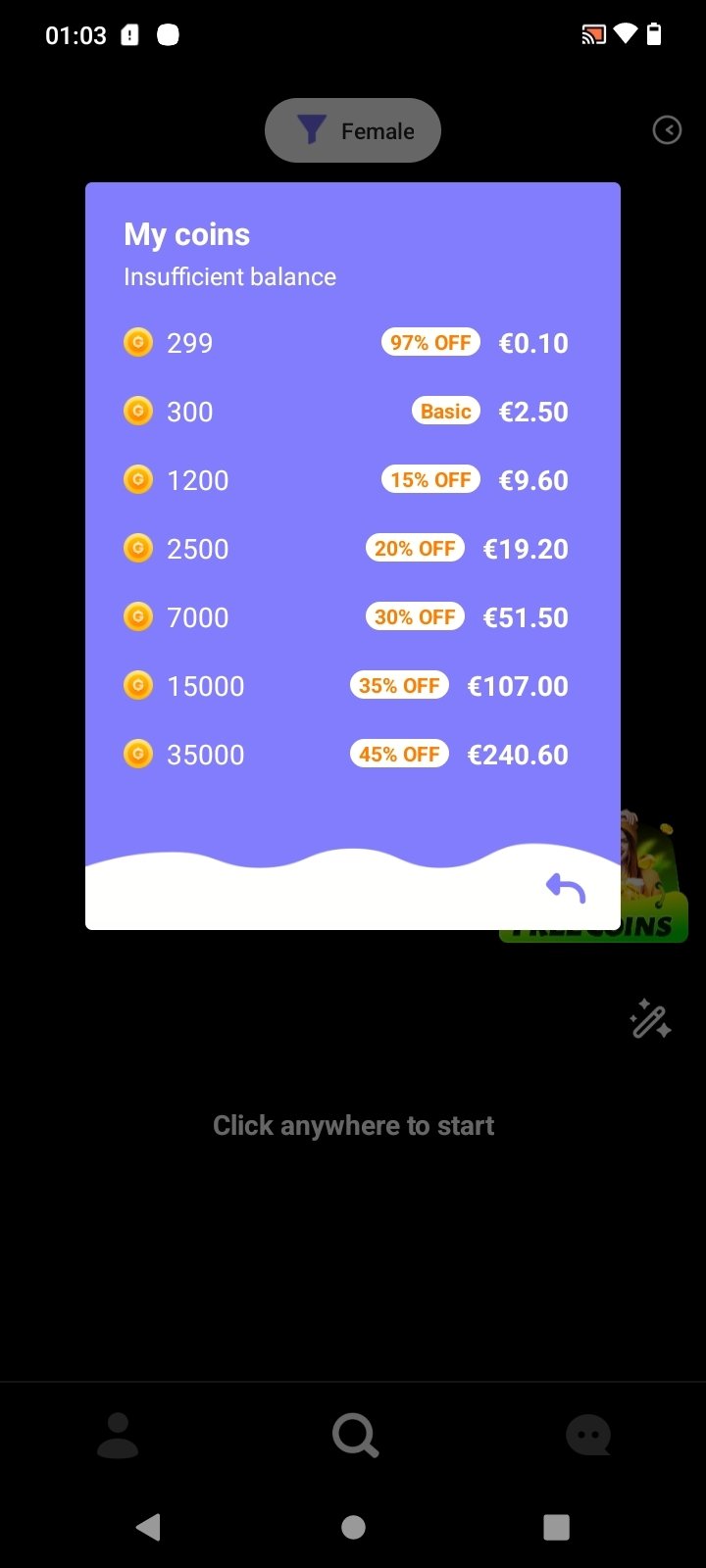The image, captured from a smartphone, depicts a promotional offer detailing various coin packages and their corresponding discounts in pounds (£). The time displayed on the phone is 1:03, and the battery is at 75%. At the top of the screen, there is an icon representing a female and another resembling a pill-shaped box. Below it, a notification reads "My coins insufficient balance."

The image lists several coin packages alongside their prices and respective discounts:

- 299 coins at 90% off for £0.10
- 300 basic coins for £2.50
- 1,215 coins at 15% off for £9.60
- 2,000 coins at 20% off for £19.20
- 7,000 coins at 30% off for £51.50
- 15,000 coins at 35% off for £107.00
- 35,000 coins at 45% off for £240.60

The background is predominantly purple, transitioning to a wavy white section at the bottom, reminiscent of a cloud. At the bottom center, it says "Click anywhere to start." There are several icons, including a search icon at the very center, an arrow shaped like a triangle, a circle, and a square at the bottom left. The screen also shows blacked-out areas, a human outline, and a speech bubble icon.